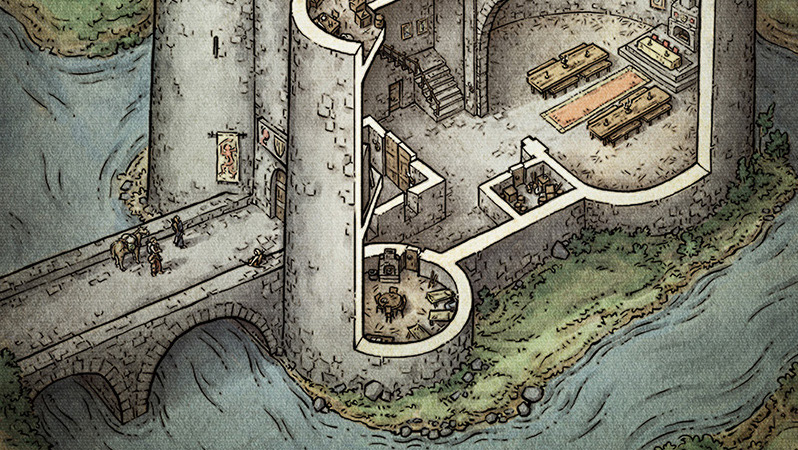This is a detailed cutaway illustration of a medieval castle, depicted from an angled, top-down perspective. The castle is surrounded by a blue-water moat, which is crossed by a stone bridge on the left side featuring two arches. The base of the castle is green with rocks, dirt, and bushes scattered around. At the front, next to the moat, there are two turrets flanking a wooden gate. A banner with a design of a red man hangs near the gate.

The castle's interior is visible due to the cutaway design. One of the turrets contains a round room furnished with beds, a table, and a fireplace. Adjacent to it, there is a small rectangular storeroom filled with brown boxes. At the rear of the castle, a staircase ascends to the left, with a door situated beneath it. On the right side is the main chamber of the castle, characterized by a grand hall setup.

This main chamber features brown tables adorned with candelabras, a red rug with a gold outline dividing them, and at the far end, a two-stepped dais. On this dais is a long table covered with a gold tablecloth, more candelabras, and three red chairs. Behind this table, a large fireplace with a log awaits the assembly. Among the architecture, two pictures decorate the wall, adding to the room's medieval ambiance.

On the bridge heading towards the castle are three characters: one person sitting on the edge, observing two others alongside a horse or donkey. Details of these characters are minimal beyond their positions and company. The water of the moat encircles the castle, complementing the green grass that frames the entire scene, emphasizing the castle's fortified nature within a lush, animated setting.